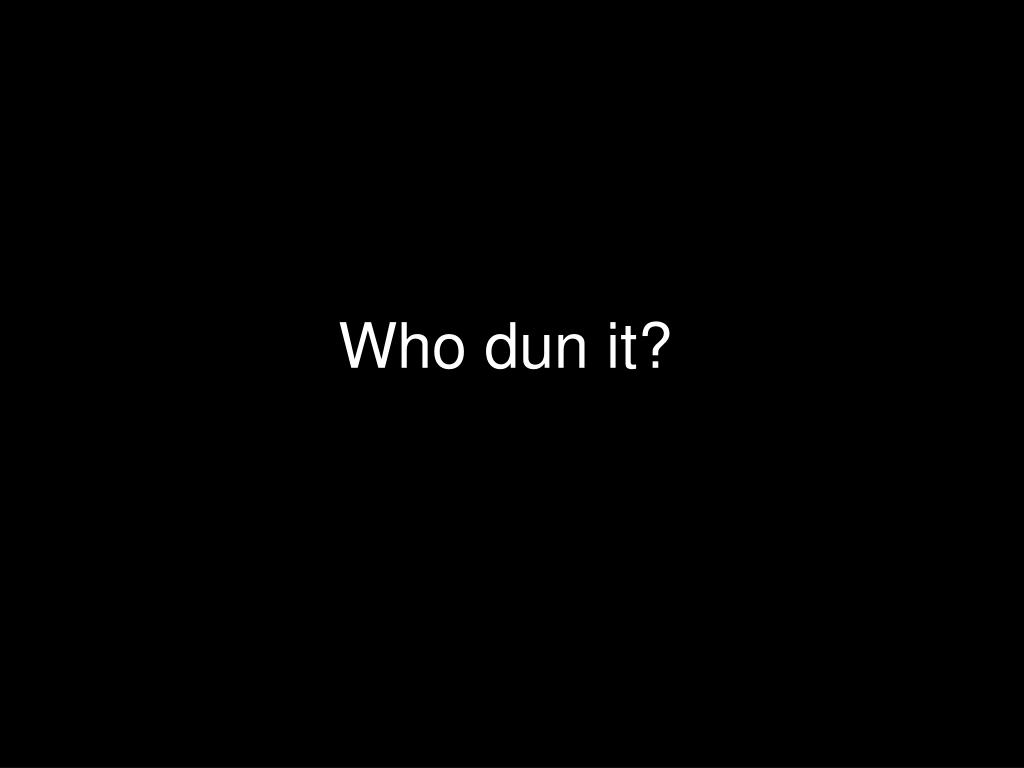The image presents a minimalist, black-and-white text with a stark and striking composition. Set against a pure black background, bold white text is centered flawlessly in the middle of the square frame. The text reads "Who done it?" — the capital W in "Who" indicating the start of a sentence, while the rest of the phrase remains in lowercase. The font closely resembles Times New Roman, emphasizing a classic feel, and the straightforward presentation gives it an almost enigmatic flavor. The phrase invokes a sense of mystery, akin to a game piece or a cue card from a mystery-solving game, reminiscent of the board game Clue. Its curious simplicity invites speculation and engages the viewer to ponder the classic question of mystery narratives.